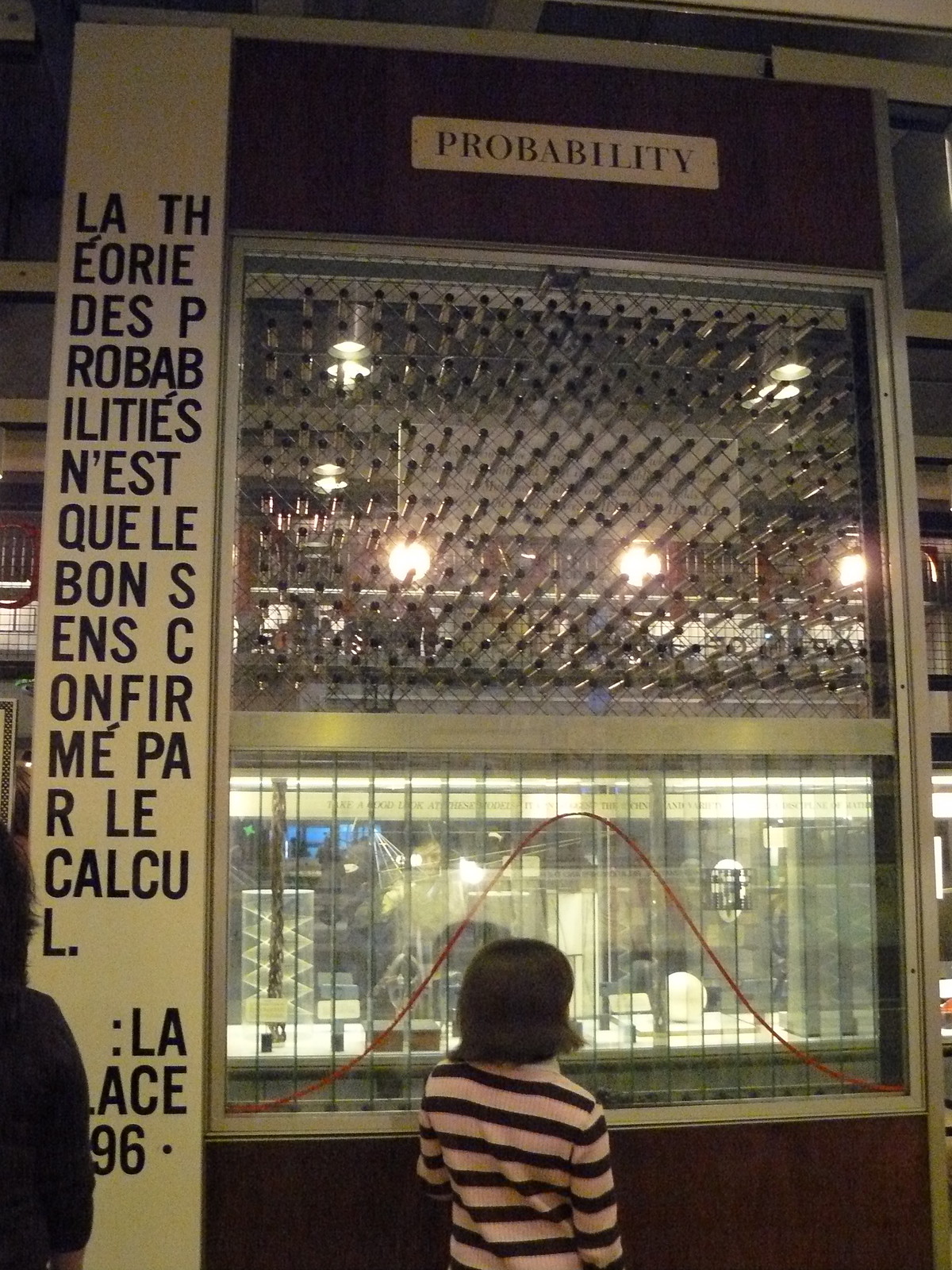In the image, a young girl with short black hair, wearing a black and white horizontally striped sweater, is gazing through a sizeable glass panel. This panel is part of the exterior of a restaurant-like building, possibly in Vietnam or another Asian country, as indicated by the challenging-to-decipher text. Above the glass window, a sign prominently displays the word "PROBABILITY" in all capital letters. The window, marked with a red line traversing from the lower left corner up to a peak and down to the lower right corner, provides a view of an interior filled with various gizmos and gadgets, and some overhead pipes. To the left of the window, a white pillar bears black French text stretching from top to bottom, reading "LA THEORIE DES PROBABILITES N'EST-CE QUE LES BONS SONT CONFIRMÉS PAR LES CALCULS LA AIS 96." Adjacent to this pillar stands the girl, who is further highlighted against a vividly green wall.